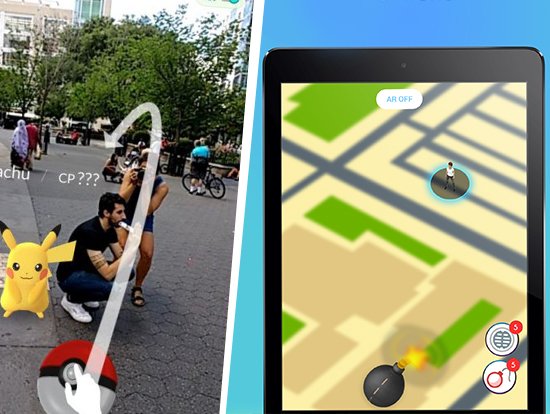The image vividly captures a lively scene where people are engaged in playing Pokemon Go against a backdrop of a bustling city park. On the left side, a man squats down, facing right, clad in a black shirt and jeans, seemingly engrossed in his Pokemon Go adventure. To his right stands a woman in a tank top and shorts, her attention also fixated on their shared game. Prominently, Pikachu appears to the left of the man, with a Pokeball positioned towards the center-bottom of the image, adorned by a curving white arrow indicating the action within the game. The right side of the image melds the real and virtual worlds, showing a street view overlaid with a bomb icon and an image of a man in a white shirt and black pants encircled by a teal ring. The phone screen displays additional game elements, including logos marked with the number five and another figure within a circle. The scene brims with the vibrant interaction of players and their game, punctuated by green bushes, trees, and the distinctive cityscape, portraying a dynamic moment of communal fun in the urban park.